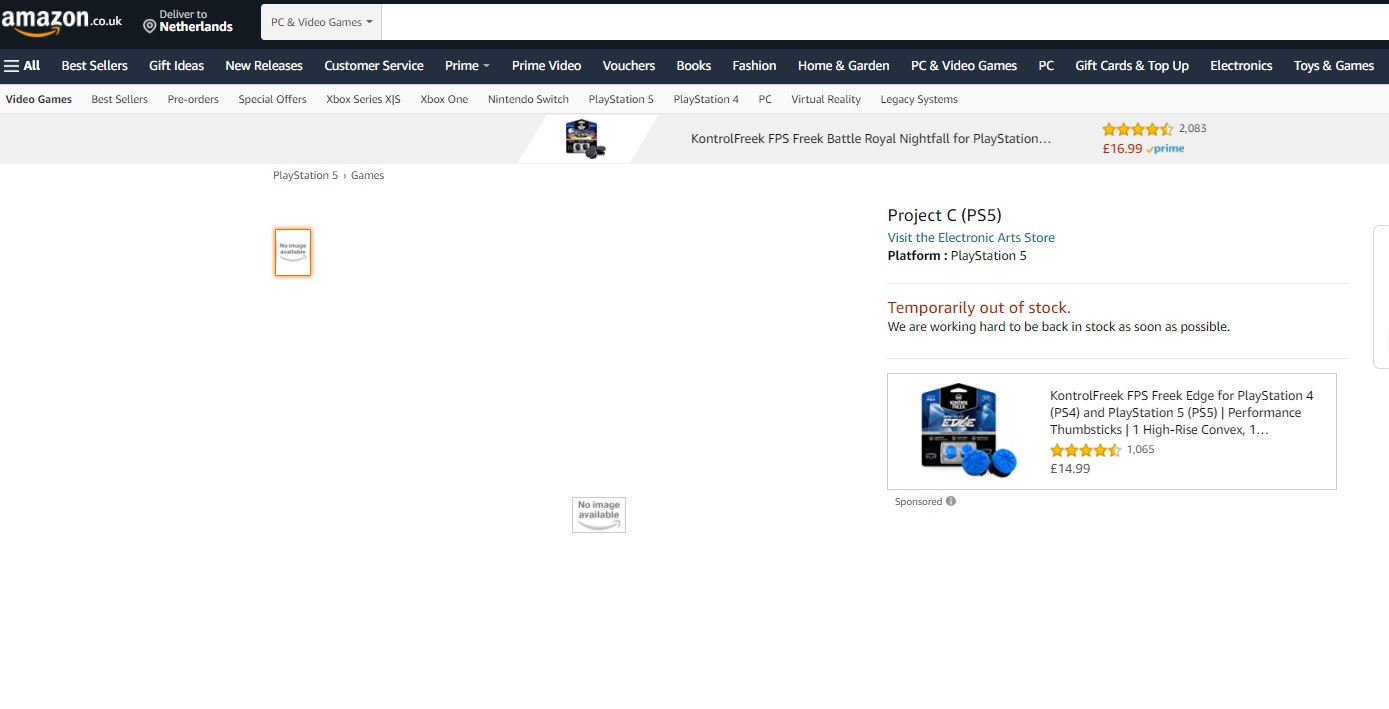In this image, we see an Amazon webpage against a white background. At the top, there's a prominent black header featuring the Amazon logo with its iconic orange swoosh and the word "Netherlands". Beneath this header, a large search bar is positioned centrally, ready for user input. 

The navigation menu below the search bar includes multiple categories: "Best Sellers," "Gift Ideas," "New Customer Service," "Home," "Prime Video," "Vouchers," "Books," "Fashion," "Home and Garden," "PC and Video Games," "Gift Cards," "Top-Up," "Electronics," and "Toys," among others.

Further down, a blue box appears with what seems to be a hard-to-read blueprint, next to which there's a small blue square. Adjacent to this is another blue box that displays a product rating of four and a half stars and a price of $16.99, indicating it's available with Amazon Prime.

Continuing down the page, we return to the white background where a small red box with white interior text is visible, and in the middle, there is another tiny box with some additional print. On the right side, the product listing titled "Project C P55" specifies its platform as "PlayStation" and notes that it's temporarily out of stock.

Lastly, there is an image of what appears to be a stylized person with large glasses, predominantly blue, with two small blue circular icons at the bottom. The product also has a rating of four and a half yellow stars.